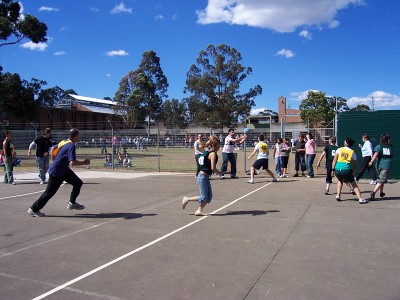This vibrant outdoor daytime photograph captures a lively scene on a cement court, possibly a playground or a basketball court, surrounded by a metal fence. The sky is bright blue with scattered white clouds, and large trees with green leaves frame the background. A dozen or so adults and possibly teenagers are engaged in an energetic game, some in motion while others wait by the sidelines. Most participants are dressed in t-shirts paired with either long shorts or jeans. A notable feature is a man towards the back clutching a blue ball, with several people focused on him. White lines are clearly painted on the court’s surface, and a tall building is visible in the distance beyond the green grassy meadow adjacent to the fence.